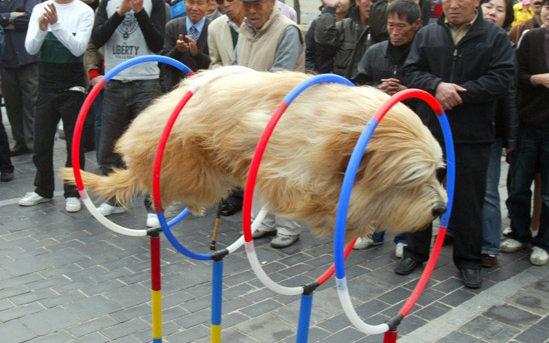In the bustling city square, a skillful dog captivates a diverse crowd with its stunning performance. The intricately trained canine leaps effortlessly through a series of suspended hoops, creating the illusion of levitating rings and baffling onlookers. Onlookers stand on ornamental pavers, their expressions ranging from sober curiosity to wide-eyed delight. The dog's horizontal dives through the hoops exude grace and precision, transforming a simple trick into an extraordinary display of agility and training. This mesmerizing scene, set against the backdrop of interested spectators, showcases the extraordinary bond between human and animal, brought to life through the artistry of pet tricks.